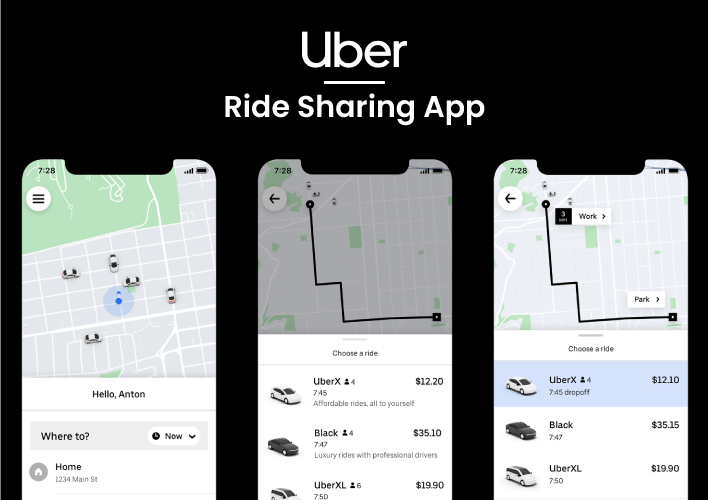This is a screenshot of an Uber advertisement characterized by a sleek black background. The focal point in the upper-middle section features the Uber logo in bold, white text, underlined for emphasis. Below the logo, the text reads "Ride-Sharing App." Dominating the center of the advertisement are three horizontally-aligned phone screen captures, showcasing different stages of using the Uber app.

The first screenshot presents a map interface with five car icons scattered around a GPS location, indicating nearby available rides. At the top, it greets the user with "Hello Anton," and includes fields to enter the pick-up and drop-off locations along with the preferred time of ride.

The second image displays a detailed route map, highlighting the path from the starting point to the destination. It also features options to select from three different ride types: UberX ($32.20), Black ($35.10), and UberXL ($19.90), showcasing pricing and vehicle category choices.

The third screenshot mirrors the route map but adds labels for the starting point ("Work") and the destination ("Park"). Similar to the second image, it offers ride choices with corresponding prices: UberX, Black, and UberXL.

This advertisement effectively illustrates the user-friendly interface and functionality of the Uber app, emphasizing ease of ride selection and route visualization.